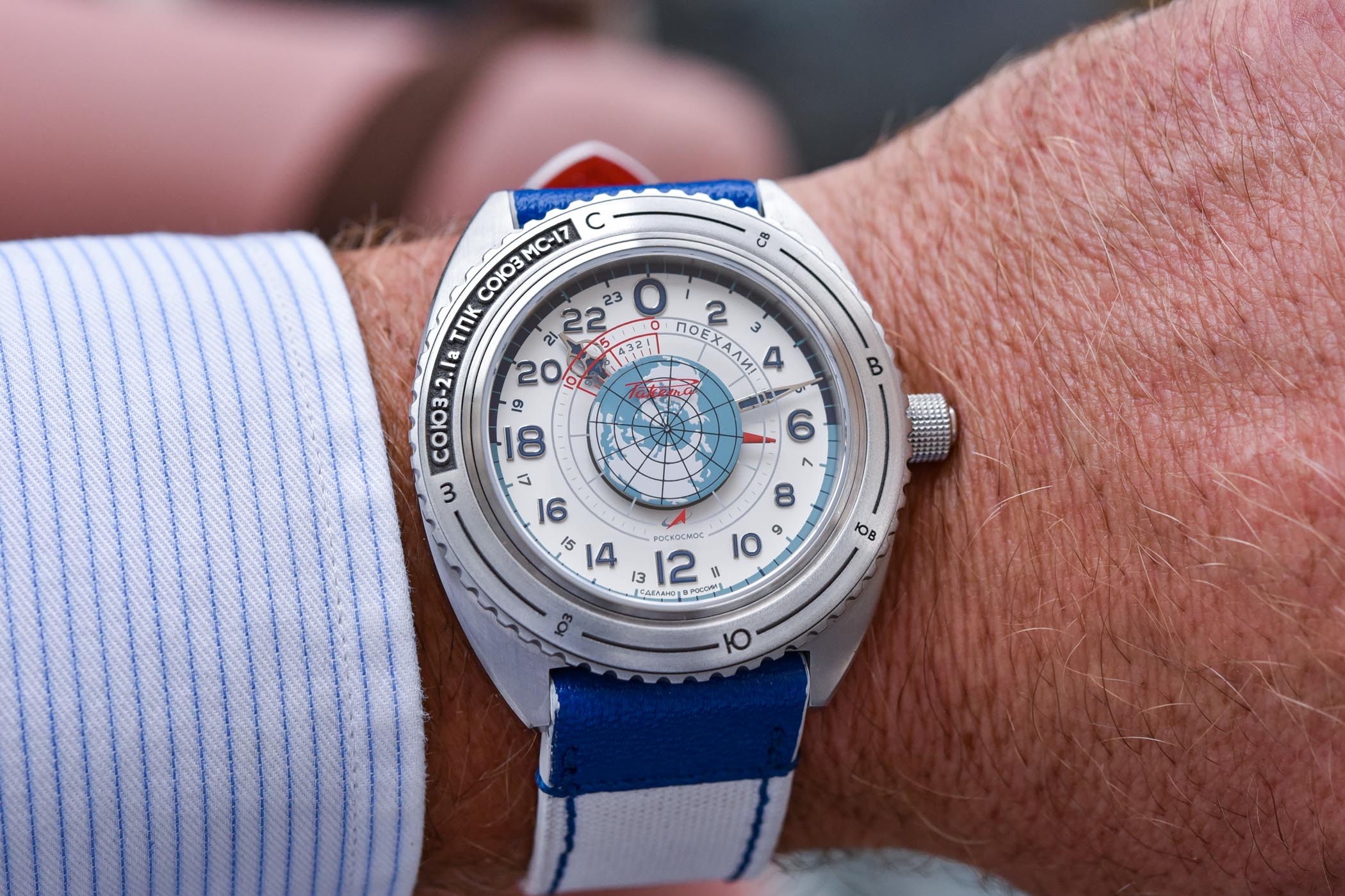The photograph showcases the wrist and hand of a Caucasian male prominently featuring a detailed wristwatch. His pale skin is covered with white or blonde hair, and he is wearing a long-sleeve shirt with thin, horizontal blue stripes like those found on college-ruled notebook paper. The watch, which stands out as the focal point, is mostly silver with a metallic sheen and features a map of the Earth in the center, overlaid with a radar symbol. It has a unique 24-hour clock face with numbers arranged as 0, 2, 4, 6, 8, 10, 12, 14, 16, 18, 20, and 22 in larger numbers, with smaller odd numbers in between. The watch also includes regular hour and minute hands, and an additional small red hand on the left side. The outer frame of the watch face is inscribed with various symbols and the text "CO 3-2-1ATNKCOL03MC-17." The strap of the watch is woven fabric in navy blue and white. The background of the image features a foggy gray backdrop with some faint pink objects, providing a contrastingly muted setting that highlights the detailed watch and the man's hand.